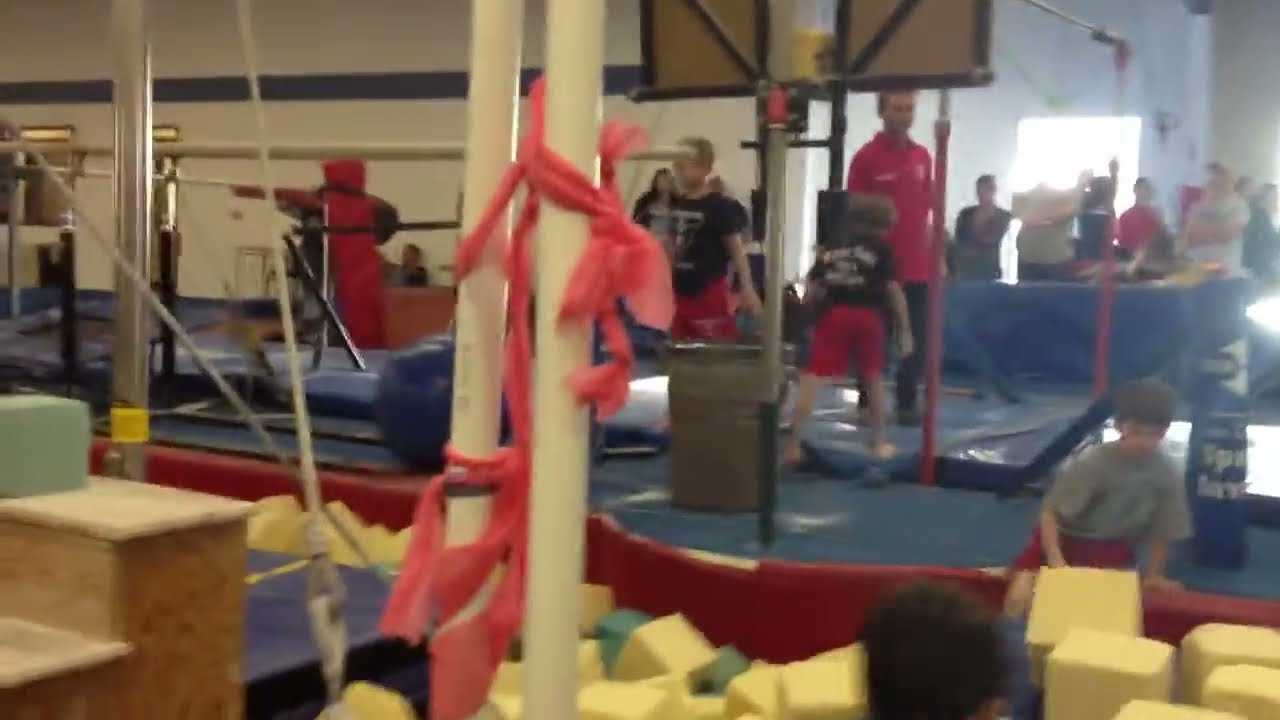The image depicts an indoor recreational facility, likely a gymnastics or play area for elementary-aged children. Dominating the scene is a large pit filled with yellow foam blocks, interspersed with a few green ones. Numerous children, about 10 to 12, are actively engaged, many wearing black shirts with red shorts that feature white writing. An adult male coach, dressed in a red shirt and jeans, oversees the activities, while other adults—possibly parents—watch from the periphery.

In the foreground, a boy around eight years old, with brown hair, is bent over reaching for a foam block. He wears a gray short-sleeved t-shirt and red shorts. Behind him, the area transitions from foam blocks to a red section, followed by a black floor, suggesting the foam pit is recessed.

The play area is equipped with various gymnastics apparatus, including blue mats, and possibly a pommel horse. Cream-colored support poles with light red fabric tied around them are situated centrally. On the left side, wooden steps, likely movable exercise equipment, add to the setup.

The background features a beige wall with decorative brown strips. Exercise equipment, such as a treadmill, is visible on the upper left, contributing to the multifunctional use of the space. The upper right quadrant reveals an open doorway emitting bright light, enhancing the indoor play area's inviting atmosphere. Additional people, wearing red and tan shirts, are scattered throughout, immersed in various activities.